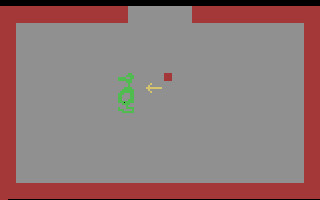In this screen capture, a black strip runs along the top edge, and a vivid red outline frames the entire display, except for a small gap, a few inches wide, right in the middle of the top section. The background is a muted gray, against which a light green figure is prominently displayed. The figure appears to resemble a rabbit, albeit ambiguously. A white arrow, pointing directly at the figure, suggests its importance or focus within the frame. At the tip of the arrow, there is a small red square, further drawing attention to this area. The context of the image is unclear, but it seems to be part of some kind of video content or graphical user interface, possibly indicating an interactive element or an instructional highlight.